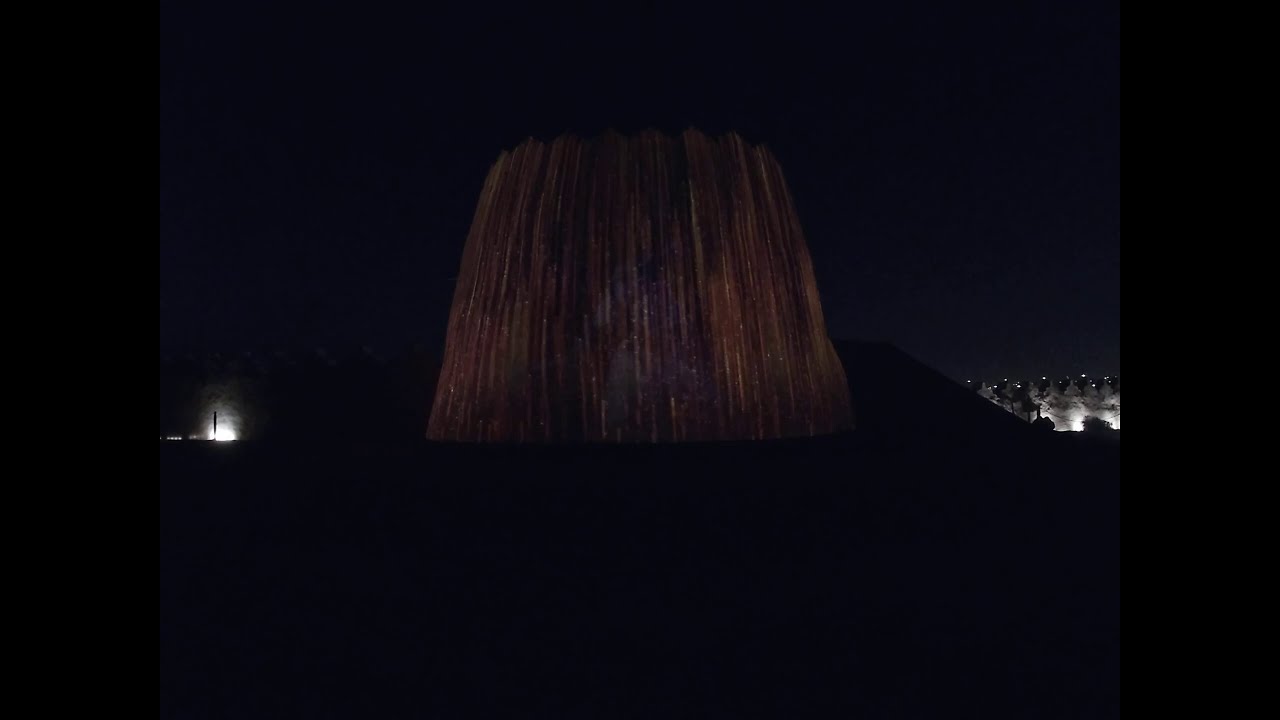This nighttime photograph captures a striking centerpiece: a large water fountain or rock formation, illuminated in a way that gives it a brownish or dark purple hue. The subject, situated in the center of the frame, resembles a plateau or a column of water with an umbrella-like shape and pointy spikes on top, evocative of a volcanic mountain or a chocolate cake. Surrounding this lit structure, the background is almost entirely pitch black, save for some faint, distant lights scattered on the left, right, and center of the image. These distant lights possibly illuminate other rock formations or small palm trees. A hint of a hill or another structure can be seen behind the fountain, adding depth to this mysterious and dark scene.